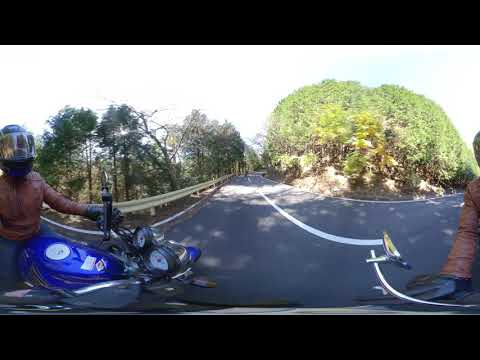In this daytime photo taken from a dash cam, the primary focus is on a bright blue motorcycle slightly turned on its side, occupying the left-hand side of the well-paved gray cement road. The motorcyclist, who is wearing a black helmet with a clear visor and a brown leather jacket, stands and turns toward the camera, though their face remains hidden due to the helmet. The road features a solid white center dividing line, and a circular gauge is visible on the motorcycle's gas tank. 

The background of the image is framed by two distinct groves of trees: darker green trees behind a guardrail on the left side and lighter green trees with a full canopy on the right. The sky above is overexposed, obscuring any view of the sun or clouds. An additional visual detail includes what appears to be the mirrored arm of the same motorcyclist wearing the same jacket on the right side of the image, although this may be a visual effect rather than a reflection of another person. The scene suggests a peaceful, possibly rural setting, ideal for a quiet motorbike ride.